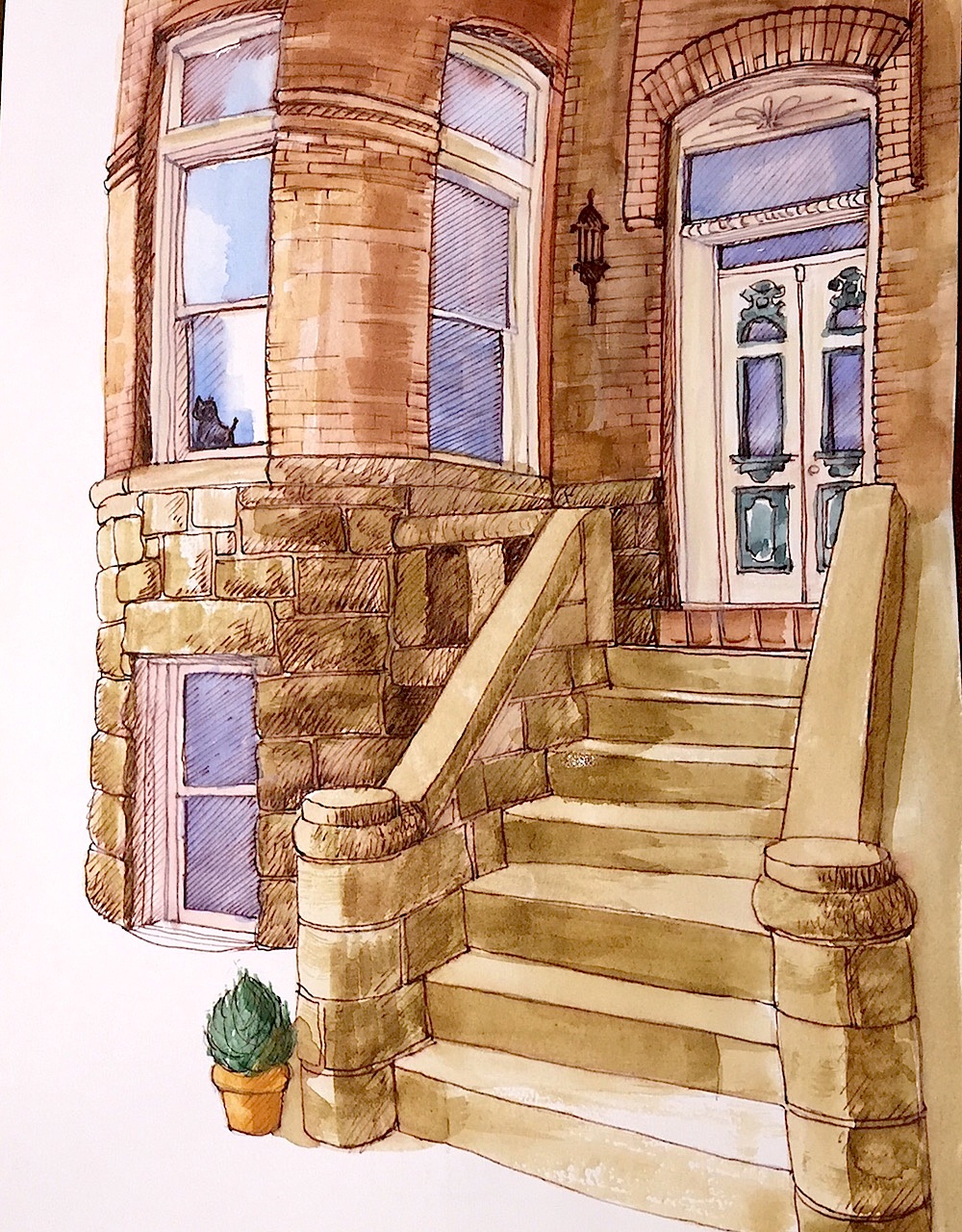This detailed illustration, seemingly from a book, vividly depicts the facade of a quintessential New York-style brick building. The scene portrays a brick exterior with elegant stone steps leading up to a double white door entrance. The doors, adorned with three small ornamental windows, open outwards. Above the door, a thin rectangular window adds to the charm, complemented by another window nestled within the arched doorway's recess.

Further up, a protruding brick element decorates the facade, distinguishing the transition between the thinner red bricks of the upper levels and the larger, more rugged stone-like bricks at the base. The upper section features two windows, each offering a glimpse into the building's interior, while a ground-level window adds balance to the structure. Adding life to the scene, a small plant is placed beside the stairway, and a curious kitten peeks out from the window, infusing the illustration with a sense of warmth and homeliness.